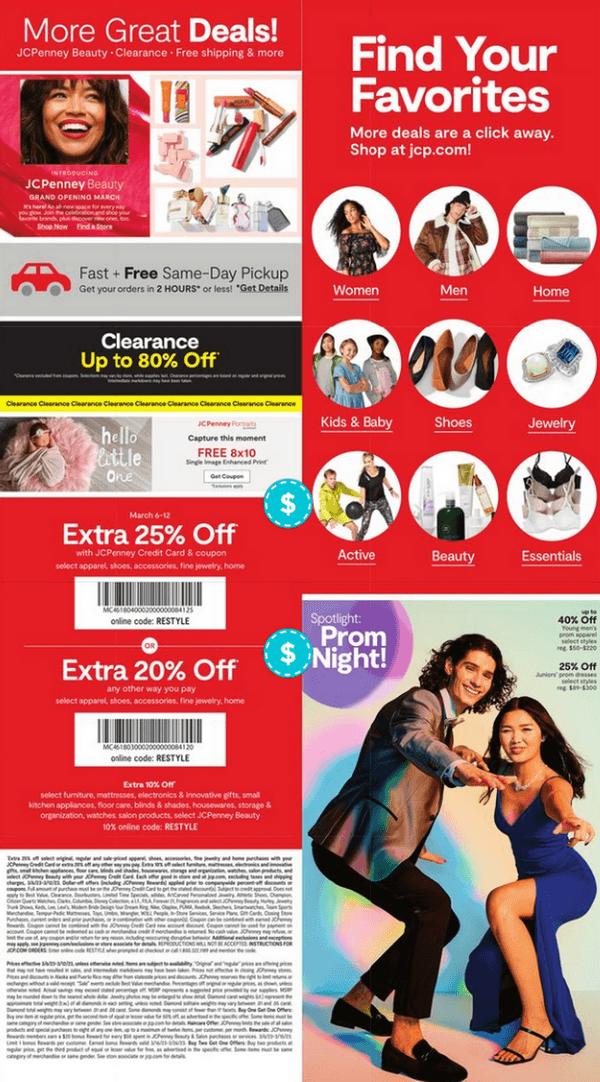**Advertisement for JCPenney: Embrace the Spotlight**

The advertisement boasts a vibrant red background adorned with bold white print, creating an eye-catching contrast. Dominating the lower left-hand corner, a white square with sleek black typography is filled with ample text, drawing attention to important details. Adjacent to this, in the lower right-hand corner, a dynamic photograph captures two spirited young individuals dancing, encapsulating the essence of joy and celebration. 

A striking purple shape in the upper left-hand corner of the photo bears the phrase "Spotlight Prom Night" in crisp white text, emphasizing the prom theme. The young man is stylishly attired in a shiny brown jacket paired with black pants, exuding confidence. His partner complements him with a pair of elegant high-heeled shoes and a flowing long blue evening gown, tastefully featuring a slit up the skirt, adding a touch of allure.

In the upper right-hand corner of the entire ad, inviting text proclaims, "Find Your Favorites. More deals are a click away. Shop at jcp.com." This section is enhanced by nine circles denoting various shopping categories, ensuring a comprehensive browsing experience. The upper left-hand corner highlights additional offers with text promoting "More Great Deals," including sections for "JCPenney Beauty," "Clearance," "Free Shipping," and other enticing opportunities.

Beneath this, a radiant photograph features a smiling woman, her joy setting the tone for the ad. To her right, an array of makeup and perfume items are showcased, enhancing the allure of JCPenney's diverse product range and inviting customers to indulge in these appealing selections.